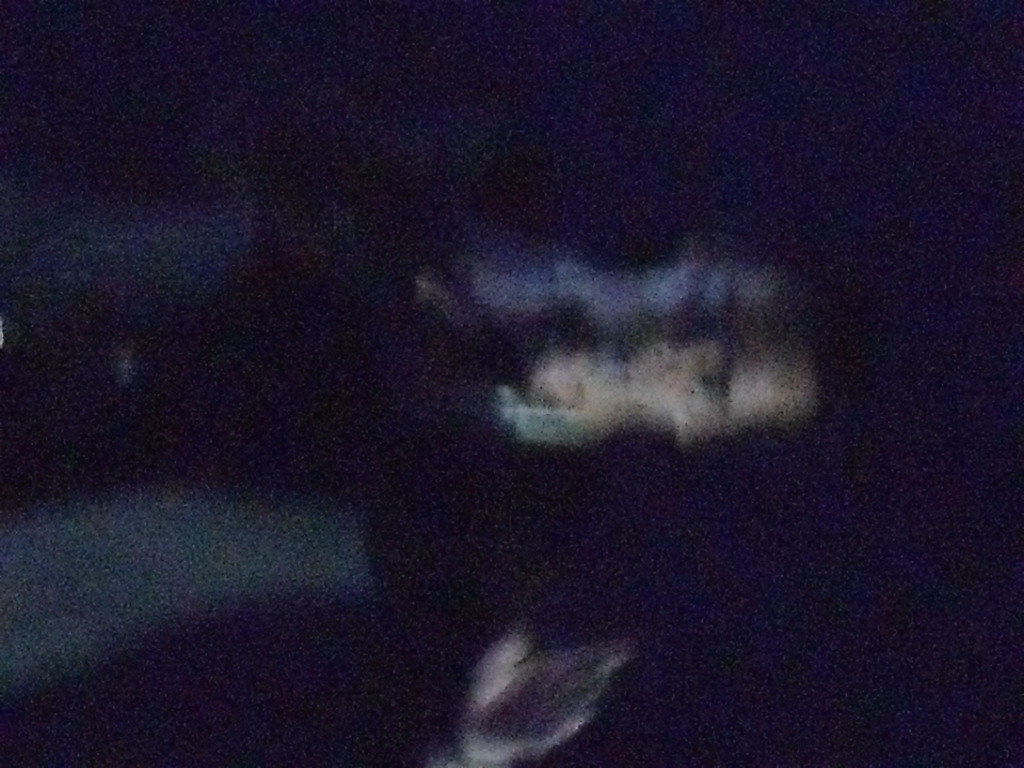This image, taken in the middle of the night, is a very blurry and low-quality photograph that appears to depict a carousel. The awning atop the carousel is faintly visible, along with indistinct shapes that resemble horses circling the structure. The extreme blurriness and potential zooming-in obscure any additional details, rendering most of the scene unidentifiable. The singular light emanating from the carousel stands out as the only source of illumination, allowing one to barely discern the subject amidst the overall darkness. Without this light, the image would be almost completely indistinguishable.